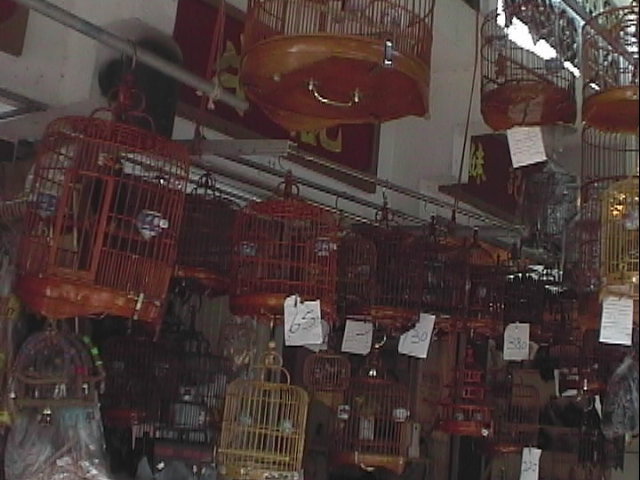The image depicts a bustling indoor market or pet store specializing in birdcages. The white-walled shop is adorned with numerous birdcages in various colors, predominantly brown, red, and some yellow or golden hues. Some cages hang from railings while others are stacked or set on stands. The cages vary in designs, with some round, metal constructions, and others resembling three-tiered houses. Each birdcage features small doors and perches inside, and many have attached white price tags ranging from $65 to $280, likely reflecting differences in craftsmanship. Hanging on the wall, there are red signs with Chinese characters, and a high window is visible in the right corner. Some birdcages hang outside the entrance, suggesting that the shop is located within an indoor market. Inside the cages, there are white and blue cylindrical cups, presumably for holding bird food.